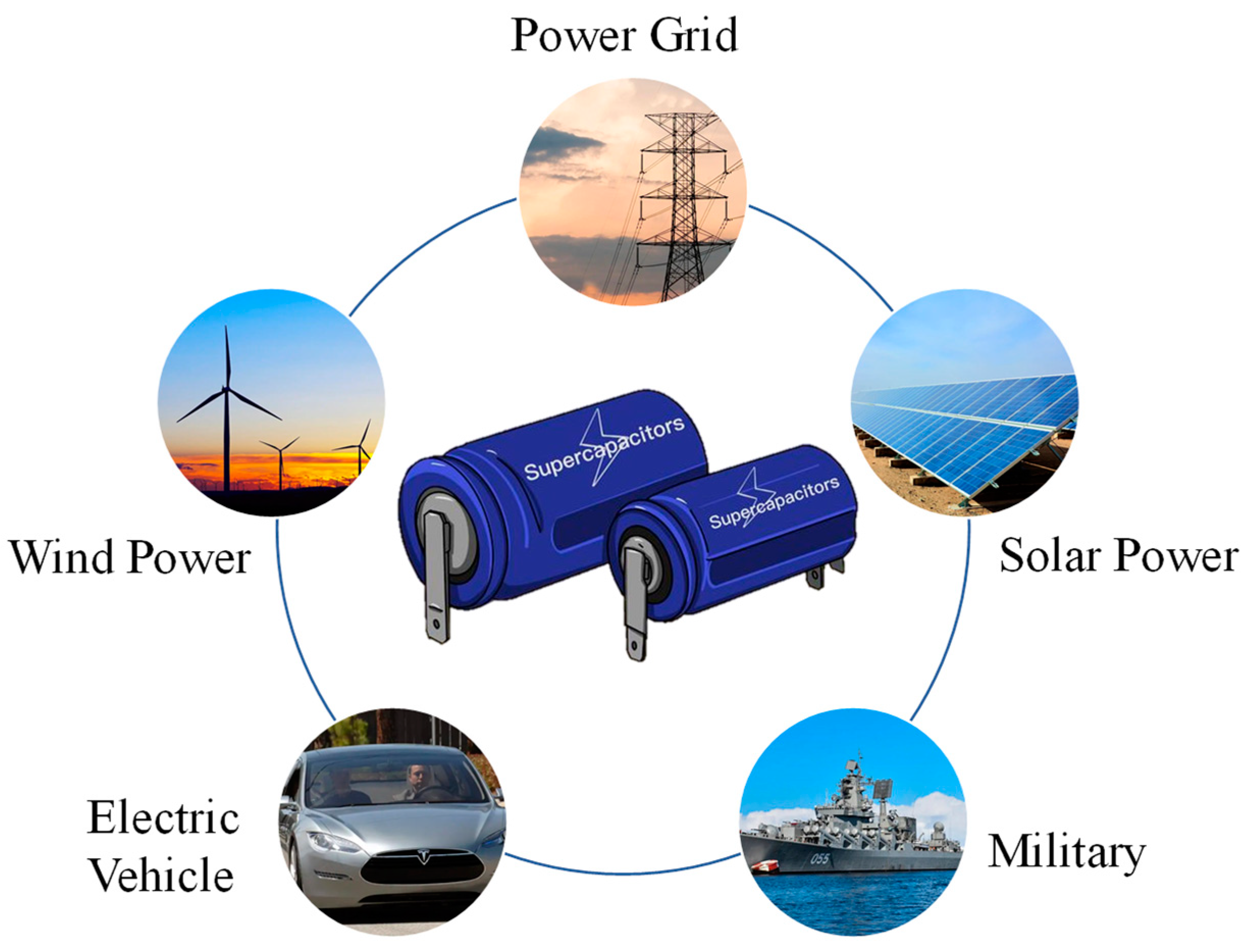The image is a detailed diagram labeled "Power Grid," featuring five interconnected circles, each representing different energy sources and applications. The first circle displays an electric line, indicating traditional electrical power. The second circle, labeled "Solar Power," shows solar panels converting sunlight. The third circle contains an image of a military warship on the ocean, marked "Military." The fourth circle features a man driving a silver electric vehicle, possibly a Tesla, labeled "Electric Vehicle." The fifth circle showcases three wind turbines set against a sunset sky, labeled "Wind Power." At the center of these circles are two blue, battery-like objects labeled "Super Capacitors," each adorned with a lightning bolt symbol, signifying their role in connecting and storing energy from these various sources.